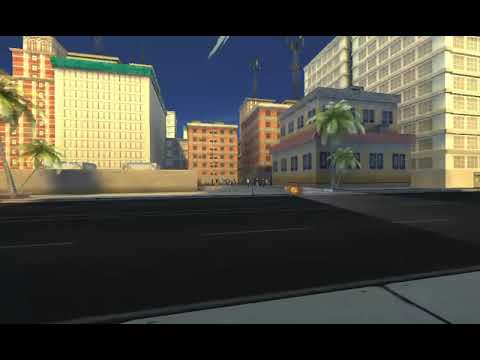The image is a detailed screenshot from a mobile or computer sniper game, viewed through the perspective of a sniper scope. The scope display is green with black crosshairs in the center. At the bottom of the scope, it reads "Distance: 200 feet," indicating the range to the target. The wind speed marker, "Wind: -20 miles per hour," is located on the right side of the scope. 

Within the crosshair view, there are two people in what seems to be a downtown area with brick buildings. One person, on the left side, wears a gray outfit and carries a brown briefcase, walking away from the scene. The other person is on the far right, dressed in a white button-up shirt and black pants, with distinctive brown hair and a beard. 

Around the scope interface, several gameplay elements are visible. On the left side, an orange "Zoom" label with an 8x magnification indicator and a slider is shown. Above this slider, there is a pause button. On the right side of the screen, icons for "Slow-mo," "Precision," and "Spotter" are displayed, along with five white bullets. These features suggest different gameplay mechanics available to the player. 

The entire scene has a 3D-rendered appearance, providing a realistic yet game-like visual of the urban environment and the targets within the sniper's view.